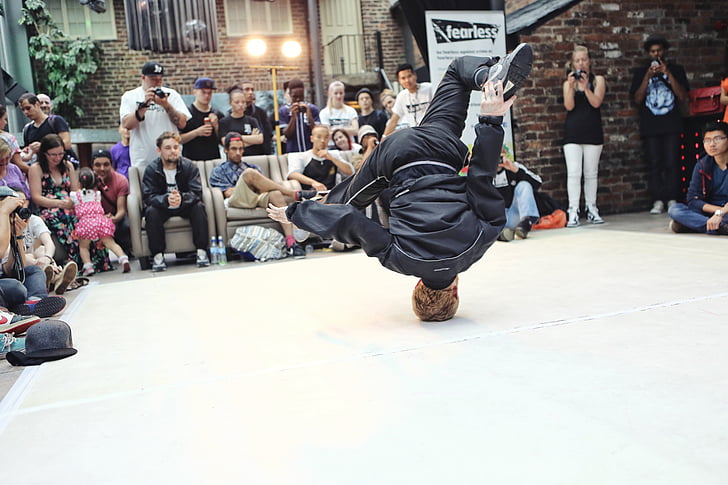This photograph captures an energetic breakdancing competition set against an urban backdrop, likely an outdoor location by a brick building with balconies and greenery peeking through. Dominating the scene, a male dancer in a black Nike jumpsuit and sneakers executes an impressive headspin on a large white mat. He strikes a visually striking pose with legs extended in a split, holding his feet with both hands. Surrounding this dynamic performance is a diverse audience—comprising adults and children—seated comfortably on grey couches and chairs, with some standing. Many are engrossed in capturing the moment with cameras and water bottles by their sides. The setting is illuminated by a pair of floodlights, and a prominent banner with the word "Fearless," along with a logo, frames the upper portion of the image, adding to the event's spirited ambiance.